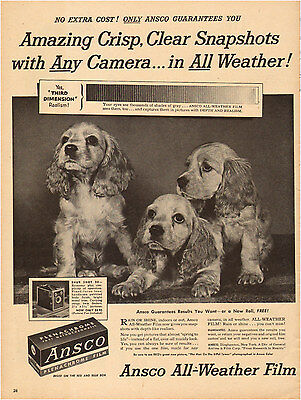This is a vintage advertisement from a yellowing newspaper or magazine, depicting an aged yet strikingly detailed page. The central image is a black-and-white photograph of three young puppies that appear to be Cocker Spaniels, reminiscent of Lady from the cartoon "Lady and the Tramp." These puppies, with their long, fluffy ears and characteristic hound dog noses, are clustered together against a dark backdrop, sitting on a floor.

The advertisement features prominent black lettering. Across the top, it reads "No extra cost! Only Ansco guarantees you amazing, crisp, clear snapshots with any camera... in all weather." Below this, a banner emphasizes "third dimension realism." There’s an image of a small black box labeled "Ansco" and a faint, blurred depiction of a camera beneath the puppies. The lower portion of the page reiterates in bold font, "Ansco all weather film." The paper's aged appearance includes tan background hues, suggesting it may have originally been white. The page number, 23, is visible in the lower left-hand corner.

This ad promotes Ansco all-weather film, promising exceptional photo quality under any conditions, capturing the compact elegance of mid-20th-century advertising.